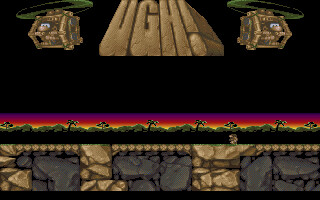This small, rectangular screen capture from an older video game showcases a vividly detailed jungle scene. The lower center of the image features a lush jungle with sporadically placed palm trees, set against a backdrop of a striking yellow and red sky. Beneath the jungle is a rock wall composed of brown and large gray stones. Dominating the center right of the wall is a discernible figure. The upper portion of the image above the skyline is pitch black. Notably, there are two helicopter-like objects piloted by monkeys, positioned symmetrically on either side of a sign that reads "UGG!" in large letters, with the sign being broader at its base than at the top. This vivid, nostalgic snapshot captures the whimsical and adventurous spirit typical of classic video games.